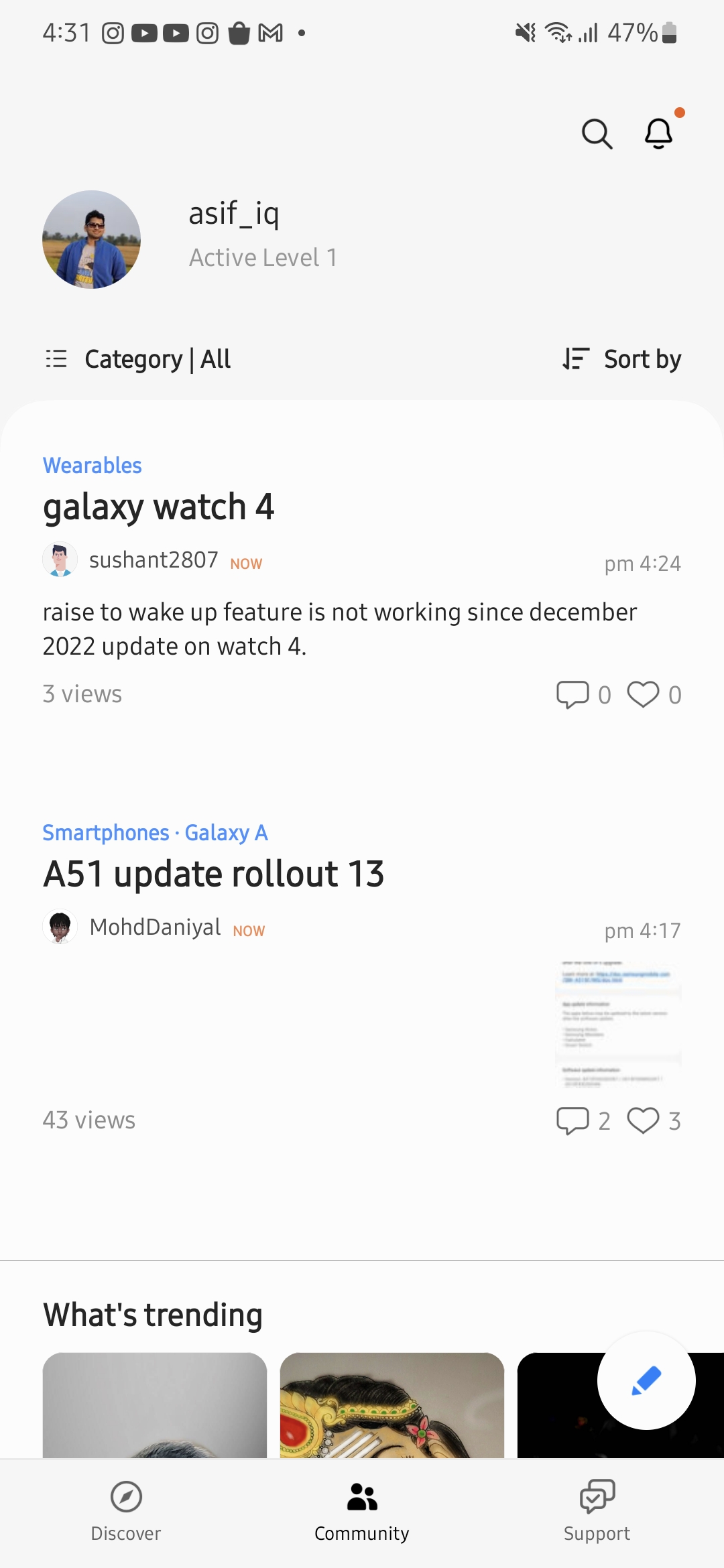Here's the cleaned-up and detailed caption based on the provided description:

---

The image appears to be a screenshot from a smartphone. The background is predominantly gray with a lighter gray section at the top displaying the time, "4:31," in black on the left-hand side. Various app icons are visible on the screen, including the Instagram logo, two Facebook logos, another Instagram logo, a gray shopping bag icon, and the Gmail "M" icon. A battery icon indicates that the phone is charging and currently at 47%.

On the right side of the screen, there is a black magnifying glass icon followed by an orange circle and a bell outlined in white but highlighted in black. Next to the bell is a profile picture of a man standing outdoors, with grass and a cloudy sky in the background. He is wearing a blue shirt and black glasses.

Beneath the profile picture, the username appears as "as_if_IQ," displayed in black text. Below the username, gray text reads "active level one," followed by the black text "category." A vertical line is drawn to separate the section on the right, which includes the options "sort by" and "wearables," written in blue. 

Further down, there is mention of the "Galaxy Watch 4" alongside the username "SUSHANT2807." A timestamp reads "4:24 PM." The text "Rise to wake up feature is not working since December 2022 update on Watch 4" is written in black, indicating an issue with the feature. The post has received three views.

Below this, the text "smartphones Galaxy A" appears in blue, and "A51 update rollout 13" follows in black. The username "MOHDDANIYAL" is listed, with the post having 43 views.

---